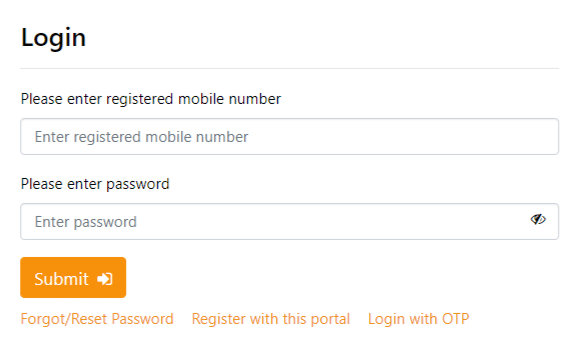The image is a landscape-oriented screenshot of a login form on a stark white background. In the upper left corner, the word "Login" is prominently displayed in dark black bold font. Directly below this, there's a thin, light gray line. Beneath the line, there is a smaller bold black instruction: "Please enter registered mobile number."

Following this instruction is a rectangular input field with a light gray border, containing placeholder text in gray: "Enter registered mobile number." Below this input field, another black instruction reads: "Please enter password."

Accompanying this instruction is a second rectangular input field with similar light gray borders and placeholder text indicating "Enter password." On the right side of this password field, there's an 'eye' icon, which, when pressed, reveals the entered password.

Further down, an orange button with the word "Submit" written in white is displayed, adorned with a red arrow pointing towards what appears to be a doorway. Below this button, three interactive links in orange provide additional options: "Forgot/Reset Password," "Register with This Portal," and "Login with OTP." These links serve as alternatives or additional actions related to the login process.